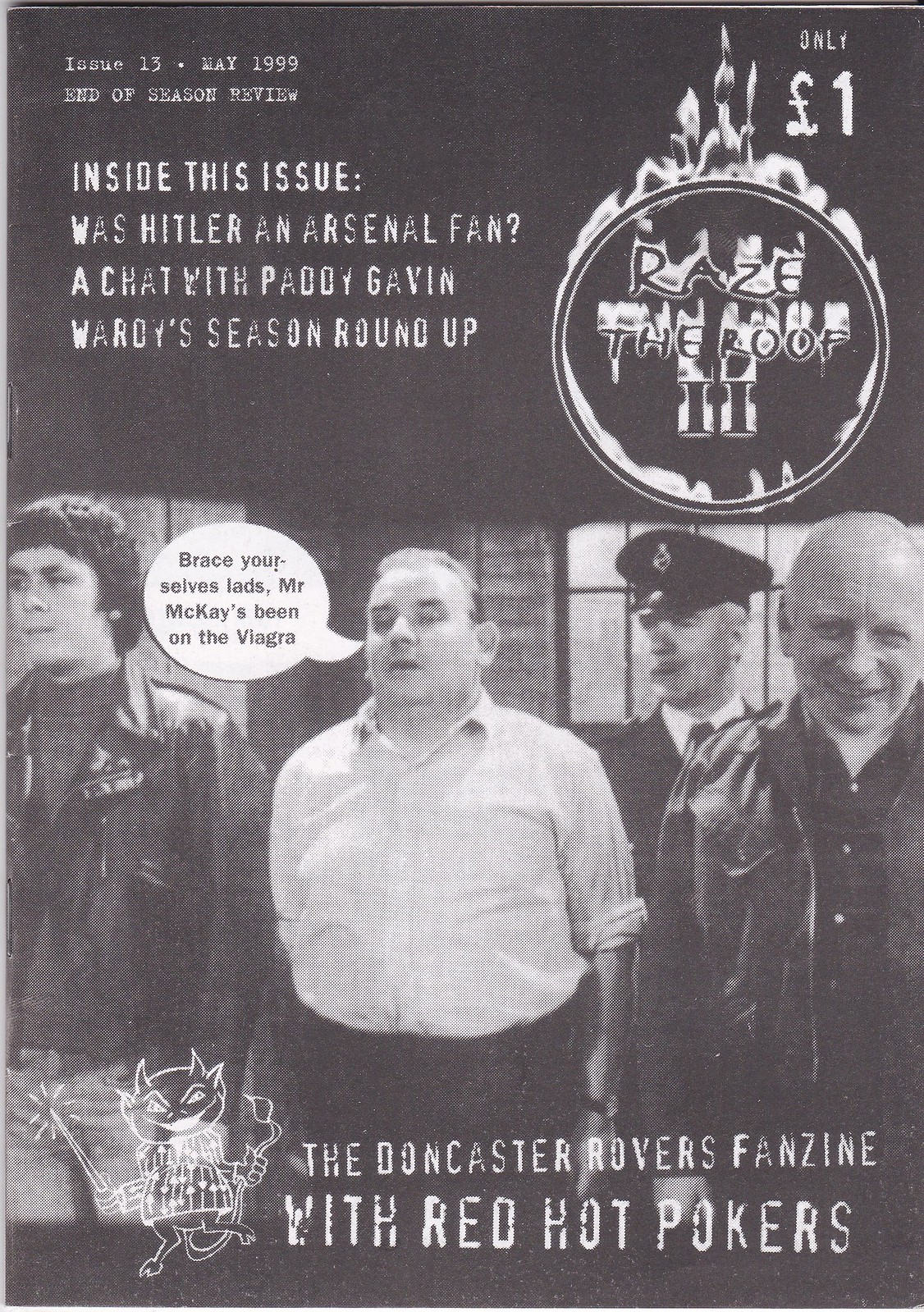This is the black and white cover of a zine, seemingly amateur-produced, titled "Issue 13, May 1999, End of Season Review." On the top right, it states the price as "Only One Pound." Prominently featuring large white text on the upper portion, the cover teases contents with, "Inside this issue: Was Hitler an Arsenal fan? A chat with Paddy Gavin, Wördy's season roundup." Below this, within a burning circular logo, it reads, "Raise the Roof II." The bottom half showcases a black and white photograph reminiscent of a TV show still, depicting a police lineup. In the center, a large man in a white shirt is being apprehended by an officer, while a bald man in a suit coat smiles at the camera and another man looks off to the left. A speech bubble over the man in the white shirt humorously exclaims, "Brace yourselves, lads, Mr. McKay's been on the Viagra." At the very bottom, a small cartoon devil holding a sword and grabbing its tail appears alongside the text, "The Doncaster Rovers Fanzine with Red Hot Pokers."